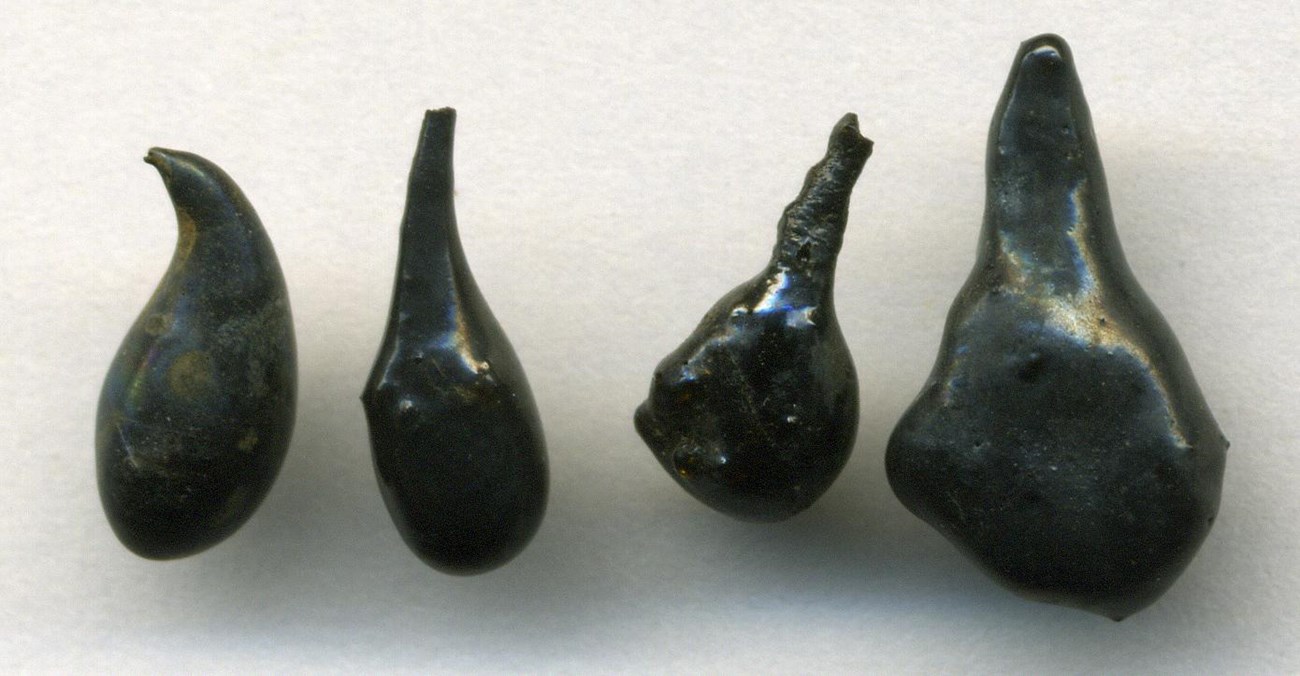In the center of a predominantly light blue background rectangle, which is wider than it is tall, there is a photograph of four dark, shiny objects that resemble small, fossilized fruits or gourds. These objects, primarily black with reflections of yellow, blue, and purple, seem preserved or replaced by minerals, giving them a polished, hard appearance much like stones or fossils. They are arrayed horizontally and vary slightly in shape and size. 

The object on the far left has an oval shape with a rounded bottom and a blunted, stem-like point that curves slightly to the left. It reflects a bit of yellow through its black surface. The second object from the left is similar but features a straighter, thinner stem pointing upwards and appears shinier. The third object is more rounded at the bottom, with a thicker, bumpy stem that has a rougher texture, though the body remains smooth and shiny. The object on the far right, the largest of the four, has a rounded base and a thicker, lumpier stem that appears less shiny and more substantial in comparison to the others.

The background transitions from light blue at the top to a darker blue at the bottom, with lighting illuminating the objects from above, casting subtle shadows beneath them. The reflective surfaces and varying textures of these mysterious objects stand out against the gradient backdrop, adding depth and intrigue to the composition.